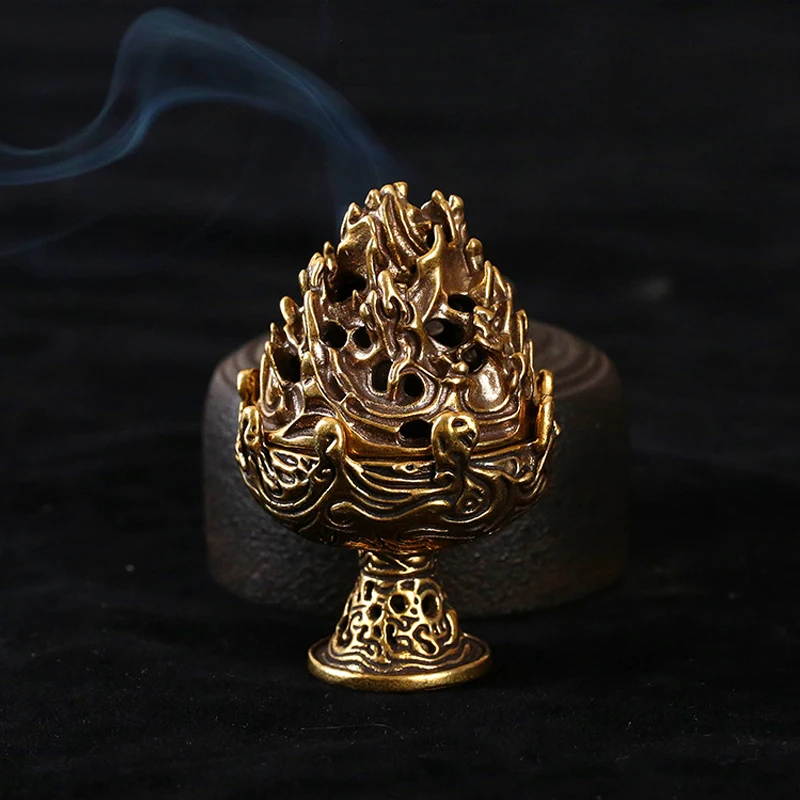Set against a stark, black background, the image showcases a detailed golden artifact that resembles a goblet or a decorative clip, adorned with intricate etchings and flowing designs. The gold-colored object, possibly gold-plated metal, sits prominently in the center, its top section reminiscent of flames or water rising upwards. Next to it is a cylindrical, brown object emitting wisps of gray smoke that drift to the left. The entire scene is illuminated with bright, clear lighting, enhancing the ornate details and professional appearance of the photograph.